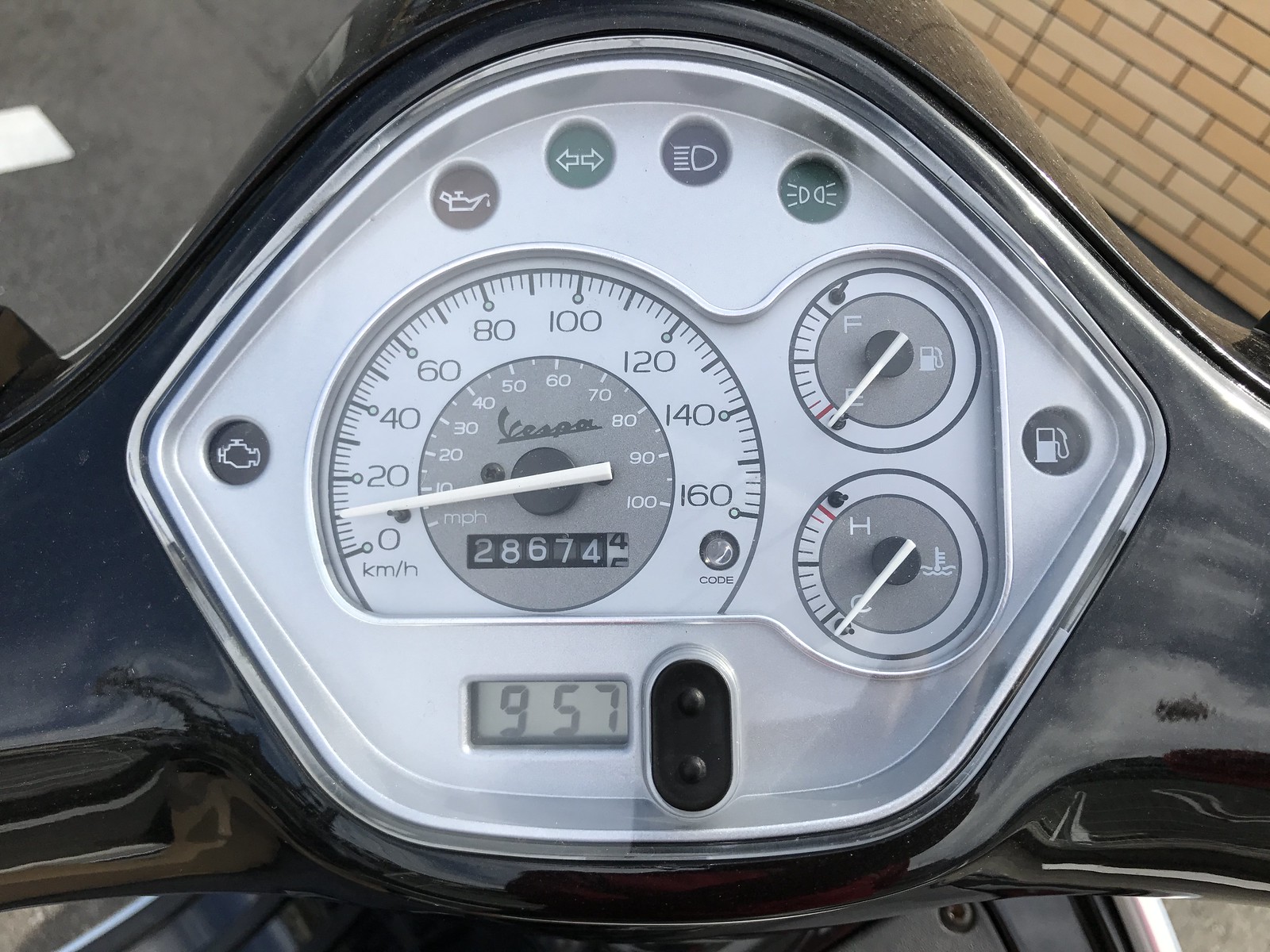A detailed close-up image of a motorcycle dashboard showcases an array of instruments and dials set against a sleek metallic background. Dominating the center is a large circular speedometer and odometer, featuring a gray center with a white dial reading 28,674 miles. Below this, a digital clock displays the time as 9:57 within a rectangular window. Surrounding the main dial, the dashboard includes smaller circular gauges indicating fuel level and engine temperature. Three dark gray indicator lights form an arc along the upper portion of the dashboard, representing various alerts including oil pressure and beam status. The background above the dashboard appears silver or white, contributing to the sophisticated aesthetic. In the upper right-hand corner of the image, a yellow brick wall with dark grouting provides a contrasting backdrop, seen at a diagonal angle. The overall composition highlights the intricate details of the motorcycle's dashboard embedded within a stylish, gray metallic framework.